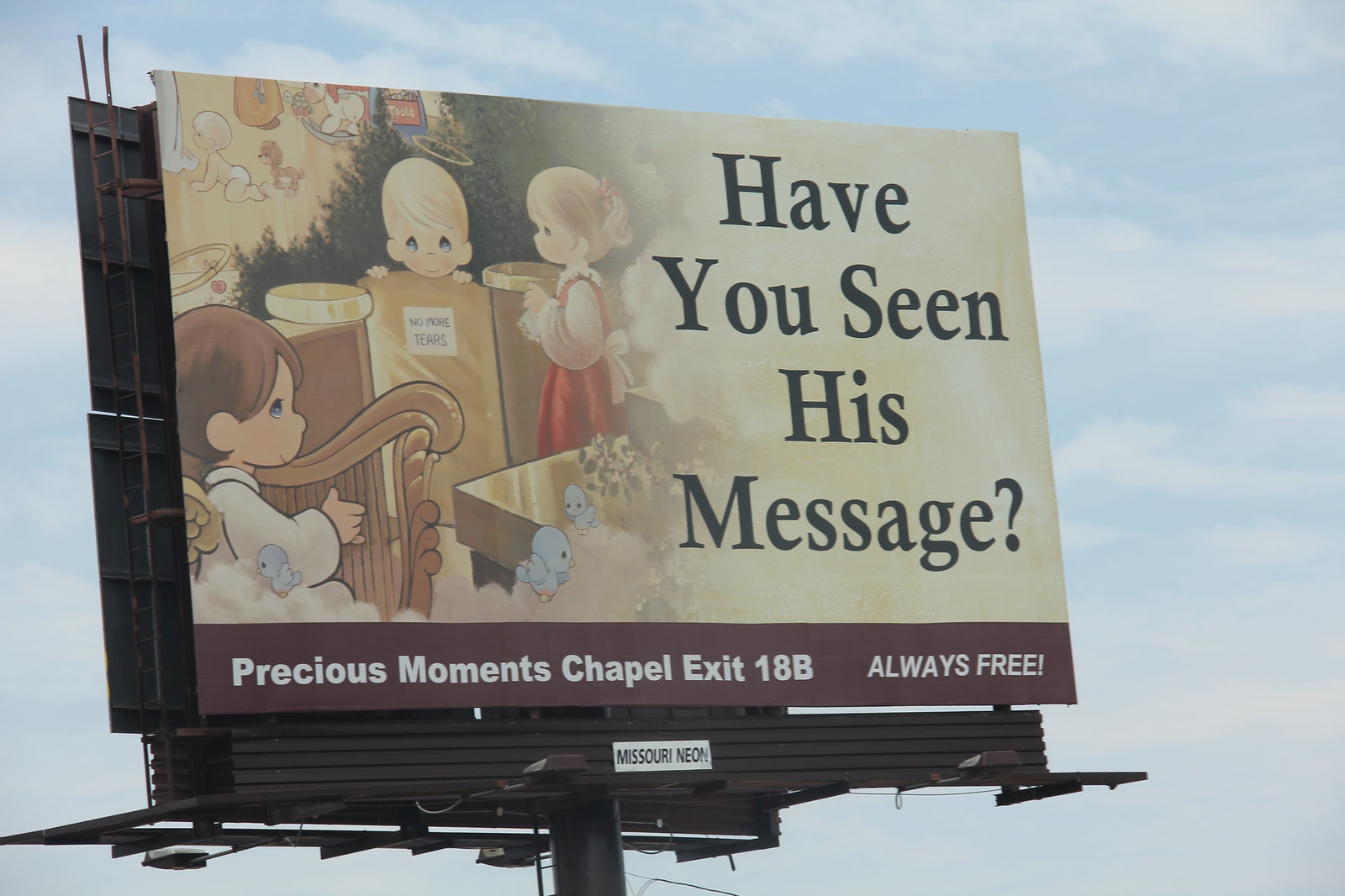This image features a large billboard set against a sky with clouds. The billboard has a tan background with the prominent text "Have you seen His message?" displayed in large letters on the right side. On the left side of the billboard, there is an illustration of Precious Moments figures.

The illustration depicts various figures, including a boy with brown hair playing a harp who has wings and a halo above his head. Next to him is a little girl with blonde hair, partially shown in profile, who is wearing a red dress over a white blouse with a white tie at the back. Additionally, a blonde-haired boy peeks over a box, next to which is a shallow bowl resting on a piece of furniture. Behind the boy is lush greenery and another halo, while the box has an unreadable message on it.

In the background of the illustration are images featuring a baby, a dog, and a rocking horse. Below the illustration, text reads, "Precious Moments Chapel, Exit 18B, Always Free." The billboard is supported against a backdrop of clouds, and it's double-sided, with another billboard visible on the reverse side.